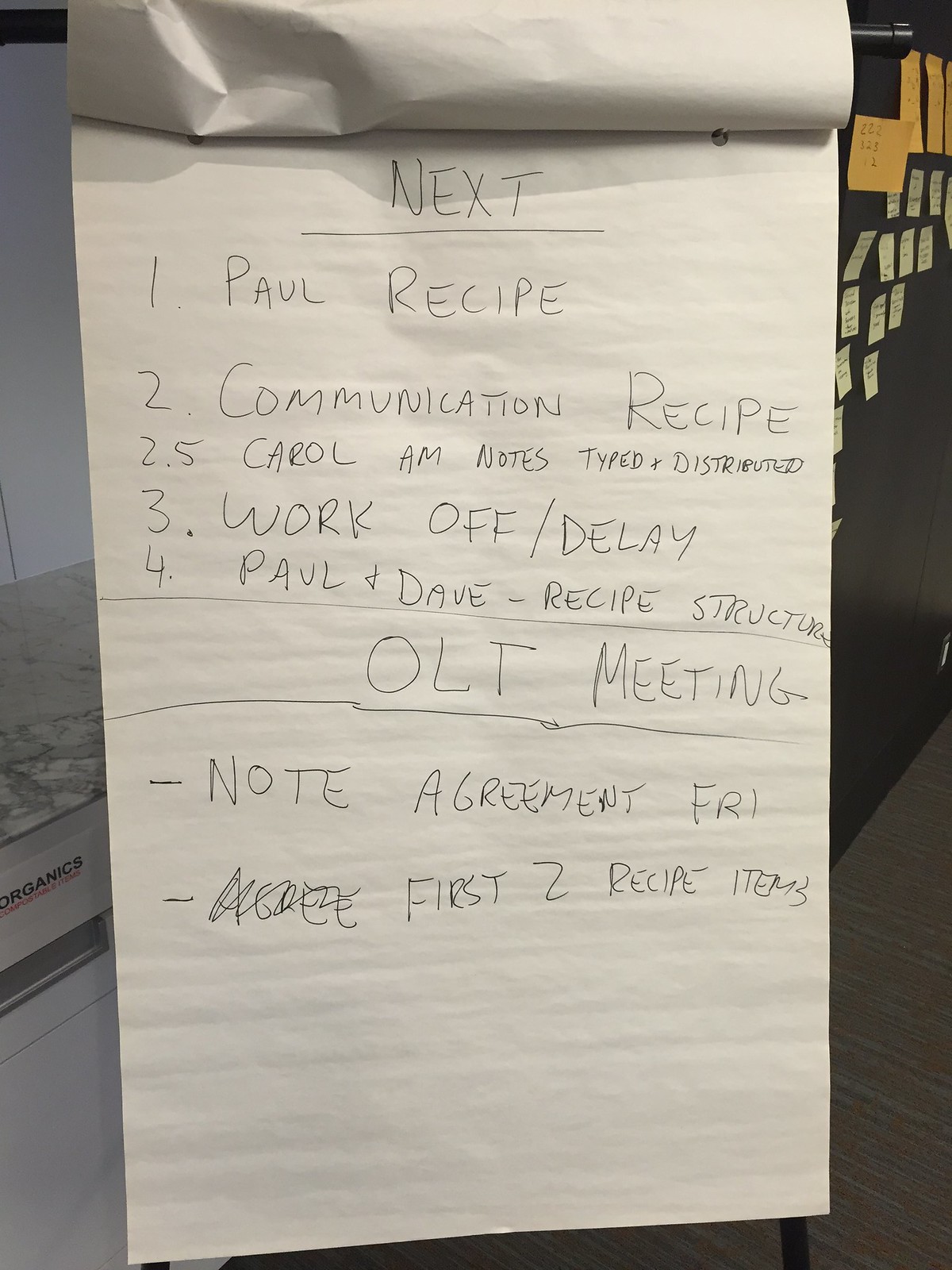The image features an open notepad displaying handwritten notes. The notes include:

1. "Next:"
2. "1. All recipe"
3. "2. Communication recipe"
4. "2.5. Carol a.m. notes typed and distributed"
5. "3. Work off/delay"
6. "4. Paul and Dave recipe structure OLT meeting - note agreement FRI - first two recipe items"

In the background, a black surface is visible, covered with numerous yellow sticky notes. Each sticky note is likely filled with additional handwritten details, contributing to the overall sense of organized planning and task management.